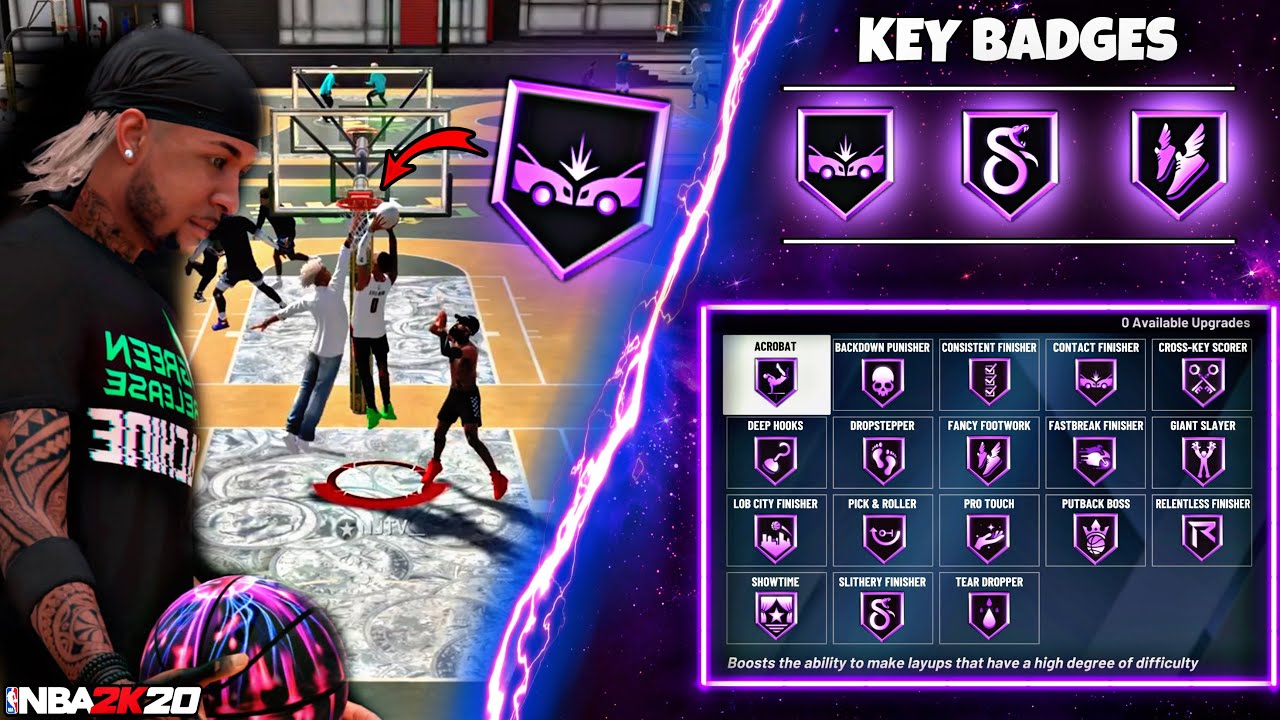Screenshot from a video game displaying the "Key Badges" section on the top right corner. Three main badges are prominently featured:

1. The first badge depicts the front view of two cars appearing to collide.
2. The second badge showcases an image of a snake, suggesting agility or a stealth aspect.
3. The third badge illustrates sneakers with small wings by the heels, symbolizing speed or swift movement.

Below these primary badges, additional badges can be seen. Some of the discernible names include "Acrobat," "Fancy Footwork," "Fast Break Finisher," "Giant Slayer," and "Teardropper."